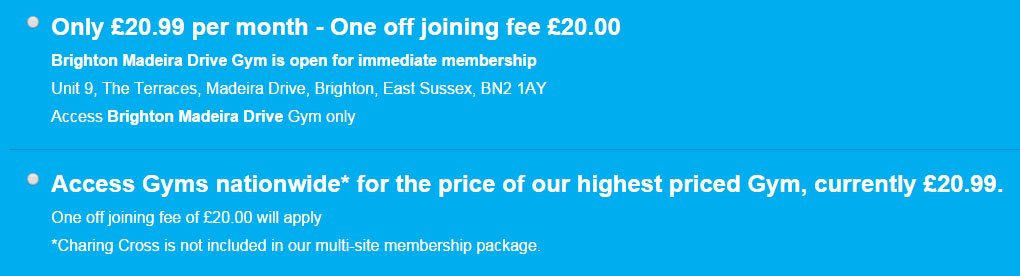This promotional image is divided into two content sections within a long rectangle shape, both featuring a light blue background. 

**Top Section:**
- In the upper left-hand corner, there is a gray bullet point.
- Next to the bullet point, a white, bold text states: "Only £20.99 per month."
- Below that, it mentions a "one-off joining fee of £20" in smaller text.
- Further down, it announces: "Brighton Madeira Drive Gym is open for immediate membership."
- The address follows: "Unit 9, The Terraces, Madeira Drive, Brighton, East Sussex, BN2 1AY."
- A bold text emphasizes: "Access Brighton Madeira Drive Gym only."

**Bottom Section:**
- A gray bullet point introduces the next statement.
- It promises "Access to gyms nationwide" with asterisk notation.
- It specifies: "For the price of our highest priced gym, currently £20.99 per month," which is consistent with the first section.
- Again, it notes a "one-off joining fee of £20 will apply", likely meaning a one-time fee.
- At the bottom, an asterisk clarifies: "Charing Cross is not included in our multi-site membership package."

This comprehensive description outlines a membership offer with specific pricing and access details, clearly indicating the details of the subscription and any exceptional clauses.